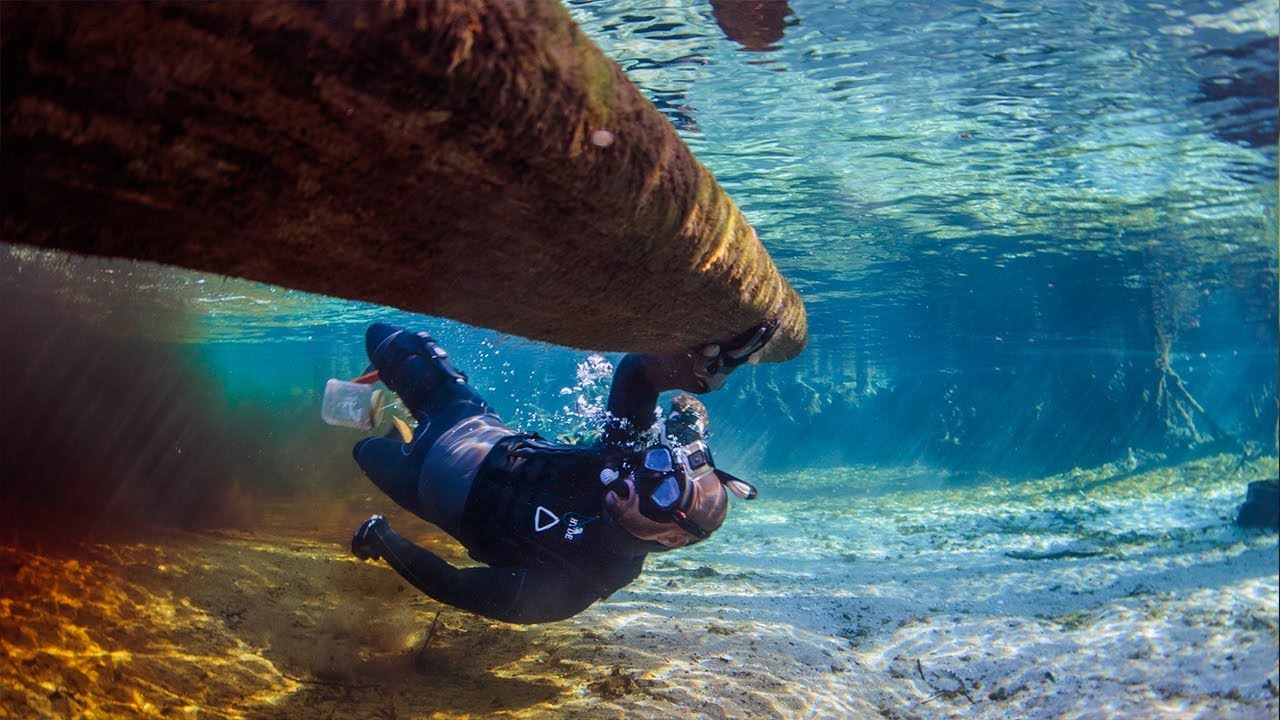This image captures an underwater scene in a shallow body of water, approximately four to six feet deep. The photograph, oriented in a landscape layout with the longer sides at the top and bottom, features a sandy bottom stretching across the frame. From this underwater perspective, the underside of the water’s surface is visible, adding a shimmering effect to the top part of the image. 

On the left side of the picture, there appears to be a ledge or perhaps the bottom of a platform or boat, extending diagonally from the upper left corner. This structure is brown and provides a contrasting element to the sandy terrain. Beneath this ledge, a diver is engaged in an activity near the seabed. Equipped with a mask and snorkel, the diver is scraping the bottom, possibly for research purposes. A sample jar is attached to a belt on the diver's leg, underscoring the scientific nature of the task. Bubbles are visibly emanating from the diver's snorkel, indicating active breathing and movement. Additionally, the submerged roots of nearby trees add an intricate network to the underwater environment, creating a rich and dynamic composition.